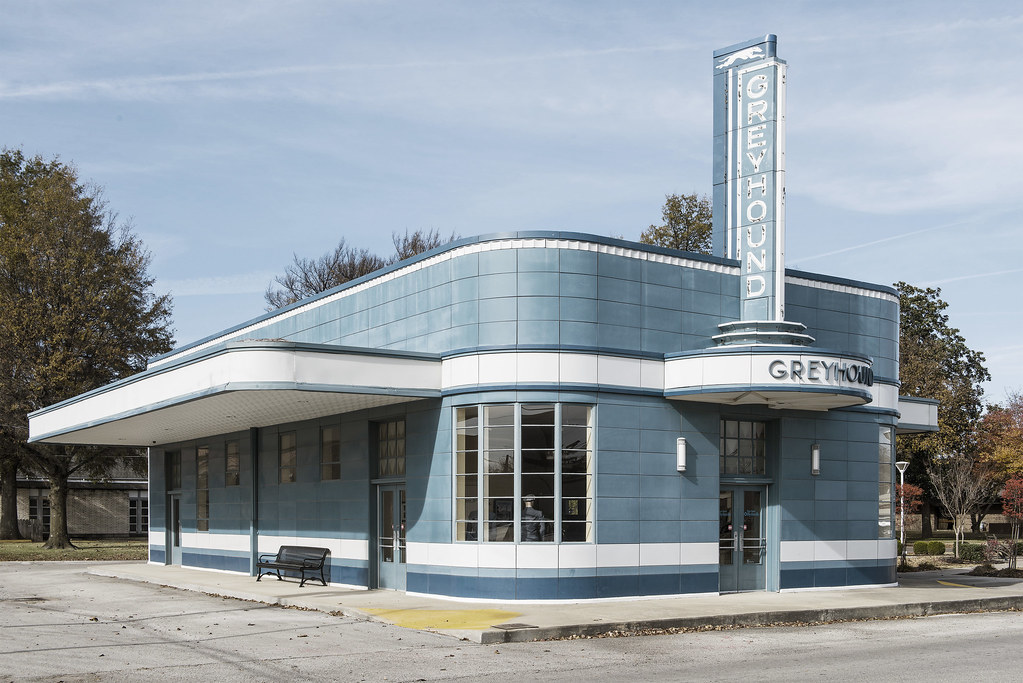The image depicts a 1950s-style Greyhound bus terminal, showcasing a design rich in period details. The building features a distinctive greyish-blue exterior with white trimmings, giving it a charming retro appeal. It has a rectangular shape with rounded edges and a flat roof. The terminal includes an overhanging area on the left side, designed for buses to pull in for boarding, and this area also shelters a black bench.

Prominently, the building's facade presents a vertical sign reading "Greyhound" with the iconic running greyhound dog logo at the top, further emphasized by a rounded white canopy portion jutting out over the doorway, adorned with three small grey knobs. The door itself, situated to the right, is flanked by lights, with a large window positioned on the left corner, offering an expansive view from inside.

The surrounding environment includes a sidewalk encompassing the front and side peripheries of the terminal, with indications of a street nearby. The day seems bright and clear, featuring a deep blue sky and some trees in the background, accentuating the serene setting of this seemingly empty yet nostalgic station. The tiles on the building's exterior are almost the same hue as the azure sky, blending harmoniously to complete the picturesque scene.